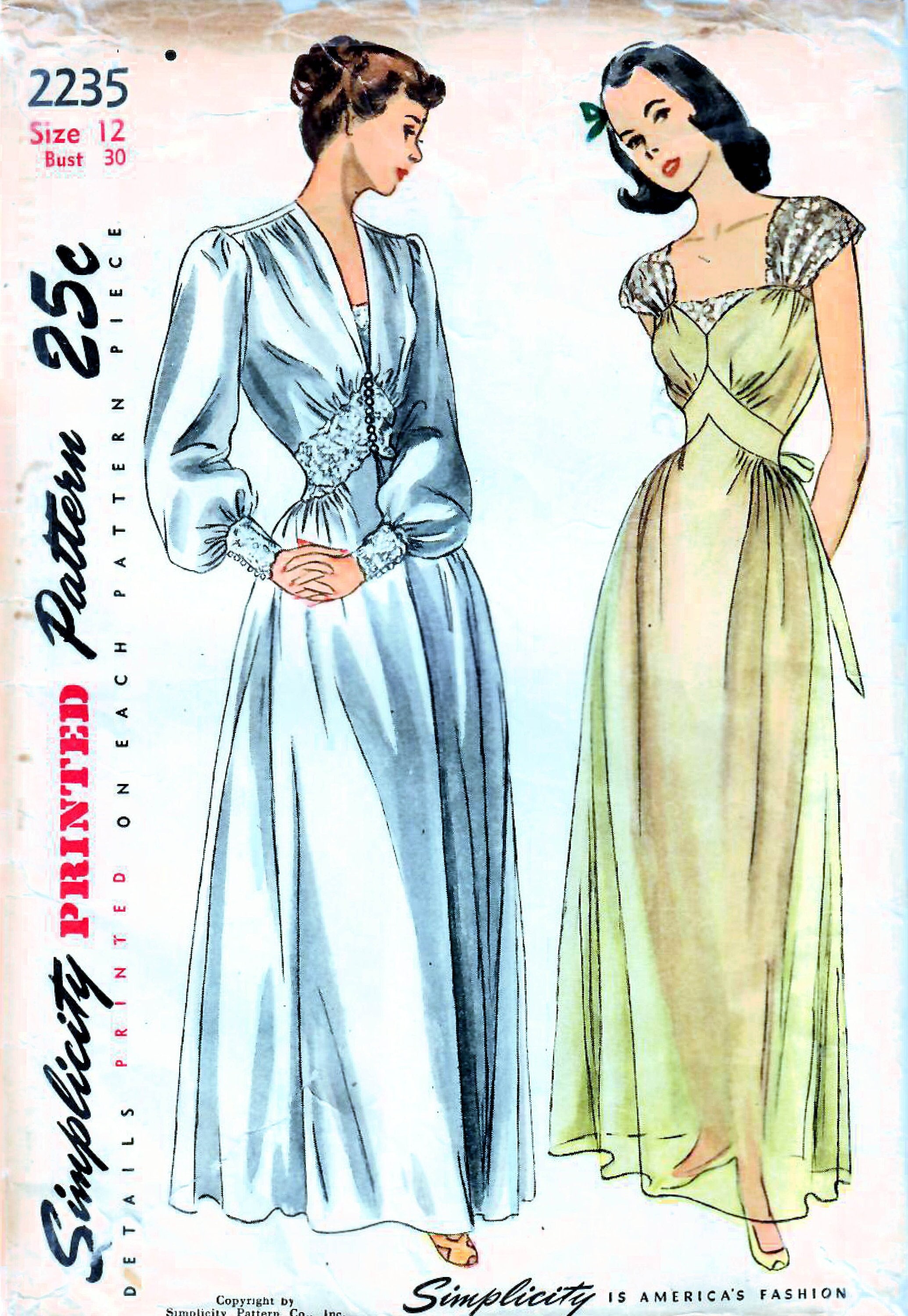This is a detailed scan of a vintage Simplicity sewing pattern, likely from the 1940s or 1950s, priced at 25 cents. The pattern number is 2235, sized for a bust of 30 inches. The image features two elegant hand-drawn women showcasing full-length dresses. The woman on the left has brown hair styled in a bun with bangs. She is adorned in a long-sleeve, deep blue gown with caper sleeves, red nail polish, and yellow slippers. Her dress is form-fitting at the waist with intricate etchings and drapes gracefully to her feet. The woman on the right, with short black hair accessorized by a green bow, dons a sheer, light green gown with mermaid-esque transparent sleeves and a bow at the back. Her dress, which flares from the waist, also reveals her legs beneath the fabric. Both women are looking to the side, the left towards her shoulder and the right somewhat towards the camera. On the left side of the image, the text reads "Simplicity Printed Pattern 25 cents. Details printed on each pattern piece," and at the top, "2235 size 12 bust 30." At the bottom, it states, "Simplicity is America's fashion."